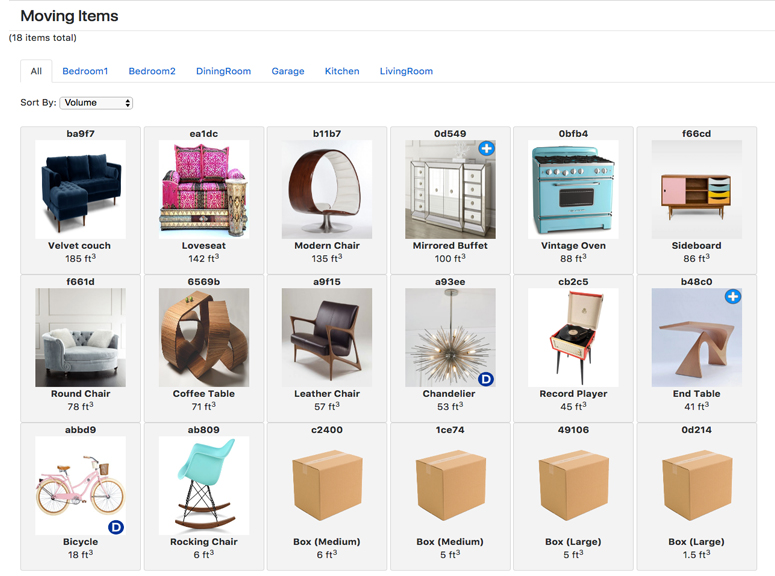Here's a cleaned-up and detailed caption for the image:

---

The displayed image is a detailed screenshot of an online storefront or inventory page, showcasing various furniture items and moving boxes. At the top left corner, the title reads "Moving Items" with a note indicating "18 items total" in parentheses. The page is systematically divided into several tabs labeled in blue font: "All" (the current active tab), "Bedroom One," "Bedroom Two," "Dining Room," "Garage," "Kitchen," and "Living Room."

Underneath the tabs, there is a sorting option denoted as "Sort by" with the current criterion being "Volume." Below this section, the page is organized into a grid of 18 squares, each representing an item. Every square contains essential details: a unique identifier or serial number at the top, a photograph of the item, the name of the item, and its volume measurement in cubic feet.

For example, the first square is labeled with the identifier "BA9F7" and displays an image of a blue couch. The couch is described as a "Velvet Couch," and its volume is listed as 185 cubic feet. The final four squares represent medium-sized moving boxes, each with its unique identifier but no specific item description, presumably for packing and transporting the other listed items.

---